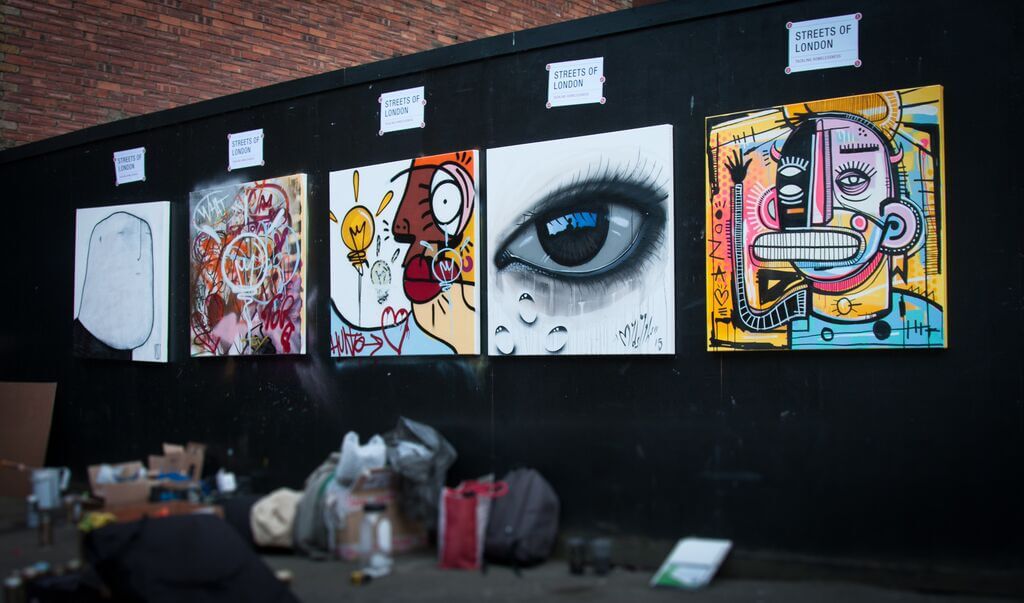The photograph captures a scene inside a cluttered indoor location with a black wall adorned with five paintings. In front of the wall, there is visible disarray with backpacks, bags, trash, and boxes overflowing with miscellaneous items, giving the area a slightly junky appearance. Above each painting, makeshift signs taped to the wall read "Streets of London." 

The first artwork, closest to the observer on the right, presents a modern, geometrically emphasized portrait featuring a being with small horns and an asymmetrical face—one side black, the other white—with a large mouth extending beyond the face's contours. Moving left, the next painting showcases a large eye against a white background. Further left, another piece carries a Picasso-like essence with abstract facial features and geometric patterns. 

The fourth painting appears chaotic, resembling graffiti with no clear form. The final artwork on the far left, presents an abstract image likened to a black and white potato. A low wall in front of the paintings partially obscures a brick wall behind, adding to the layered visual complexity of the scene.